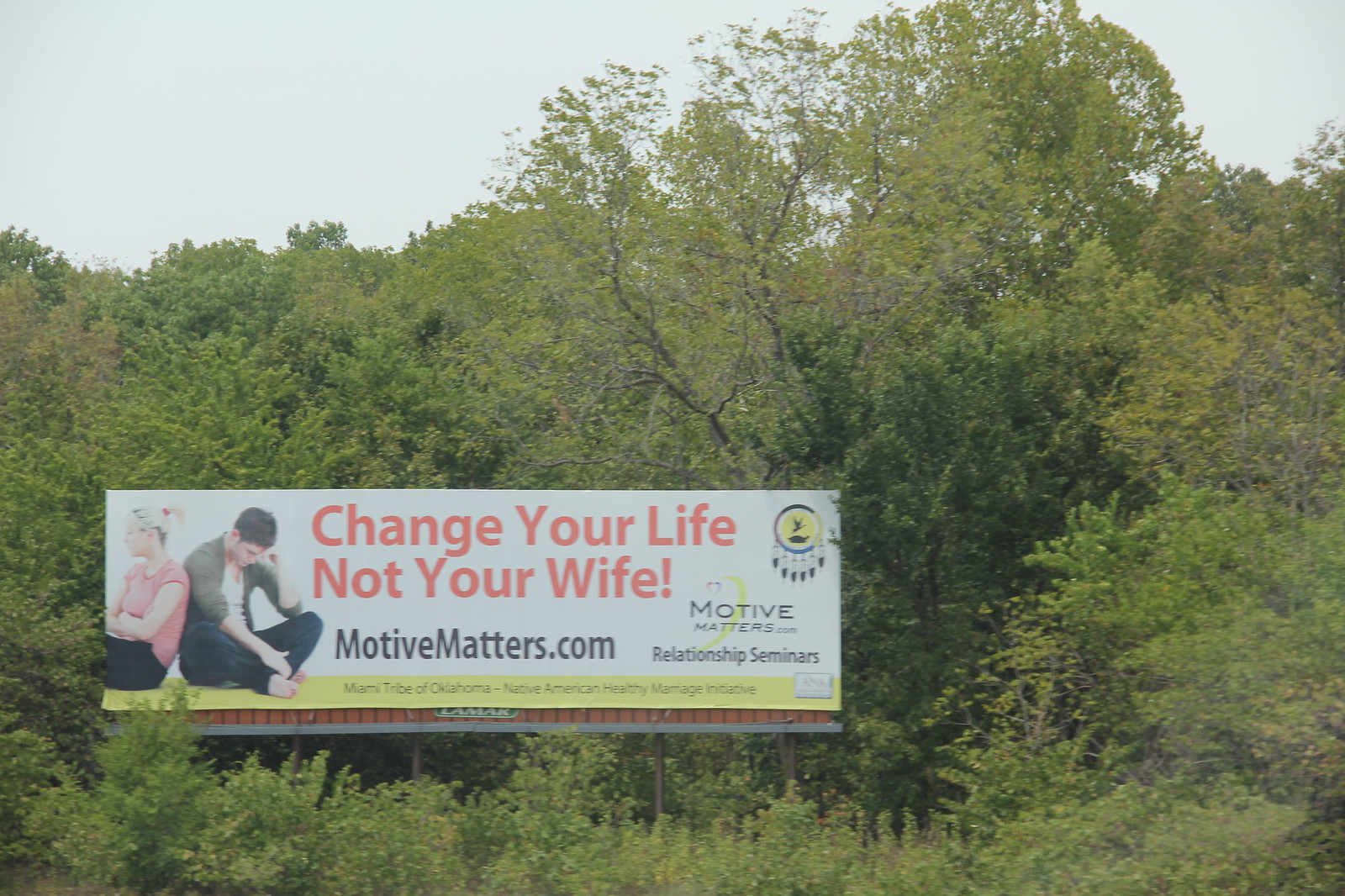The photograph captures a prominent billboard situated along the freeway, with a background of dense, leafy green deciduous trees and a cloudy, grayish-white sky. The billboard itself is white, adorned with a yellow strip at the bottom and a touch of red beneath it. It features an image of two people sitting back-to-back at the bottom left of the billboard. The female, with blonde hair tied in a ponytail, wears a pink shirt and black pants, her arms crossed as she looks into the distance. The male, dressed in a green t-shirt with dark pants and a white undershirt, has his left hand resting on his head, elbow on his knee, with his gaze angled downward. Dominating the billboard in bold red letters is the text: "Change your life, not your wife." Below, in dark letters, is the website: motivematters.com. On the right side of the billboard, the text "Motive Matters Relationship Seminars" is displayed, accompanied by an image resembling a dreamcatcher in the top right corner. A yellow band at the bottom reads, "Miami Tribe of Oklahoma Native American Healthy Marriage Initiative." Low-growing bushes obscure the base of the sign, completing the scene.